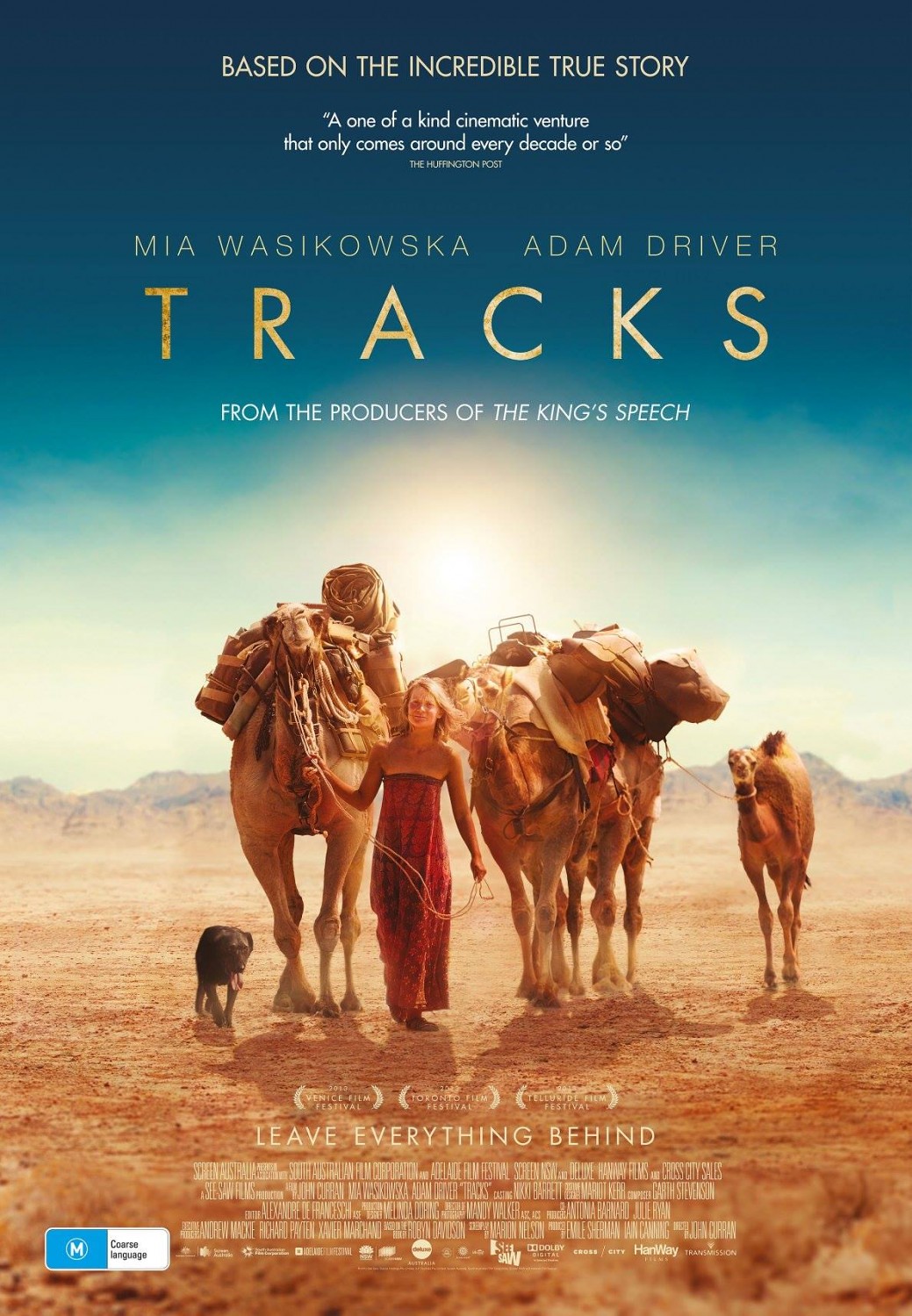This movie poster for "Tracks," headlined by Mia Wasikowska and Adam Driver, advertises a film based on an incredible true story. It features a prominent quote from The Huffington Post: "A one-of-a-kind cinematic venture that only comes around every decade or so." The poster also includes the tagline "Leave everything behind" and highlights that the film is from the producers of "The King's Speech." 

In the central image, a white woman in a red dress is depicted pulling a laden camel with a rope, while at her side are two additional camels, also heavily loaded with bags and supplies. A black dog accompanies them, walking to the far left. They are wandering in a vast desert setting. Additional details at the bottom of the poster mention accolades from the 2010 Venice Film Festival, the 2023 Toronto Film Festival, and the 2018 Telluride Film Festival. The movie is rated M, which is marked clearly in a blue rectangle at the bottom alongside various production logos such as Seesaw Films, Dolby Digital, and Transmission.